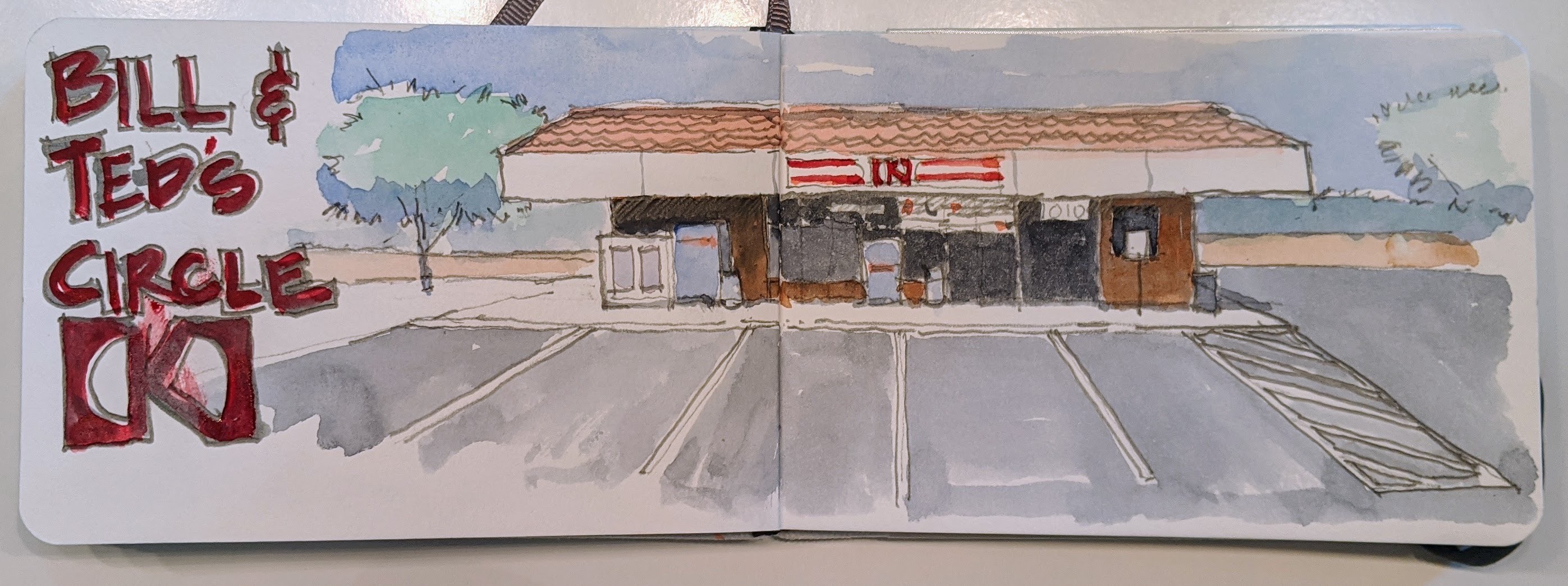This image features an artistic drawing displayed on an open portfolio, showcasing a detailed illustration of a convenience store titled "Bill and Ted's Circle K." The flat-roofed building, adorned with a brown rooftop, is situated in the center of the image within an empty, gray parking lot complete with delineated parking spaces. An ice machine is positioned to the left of the store's entrance, while signage decorates the convenience store facade, although no text is clearly readable beyond the prominent red writing on the left page that spells out "Bill and Ted's Circle K." The background includes a blue sky and two trees, one on each side flanking the building, with a road running behind the store but devoid of any vehicles. The entire scene evokes a serene, quiet atmosphere typical of small, roadside convenience stores.